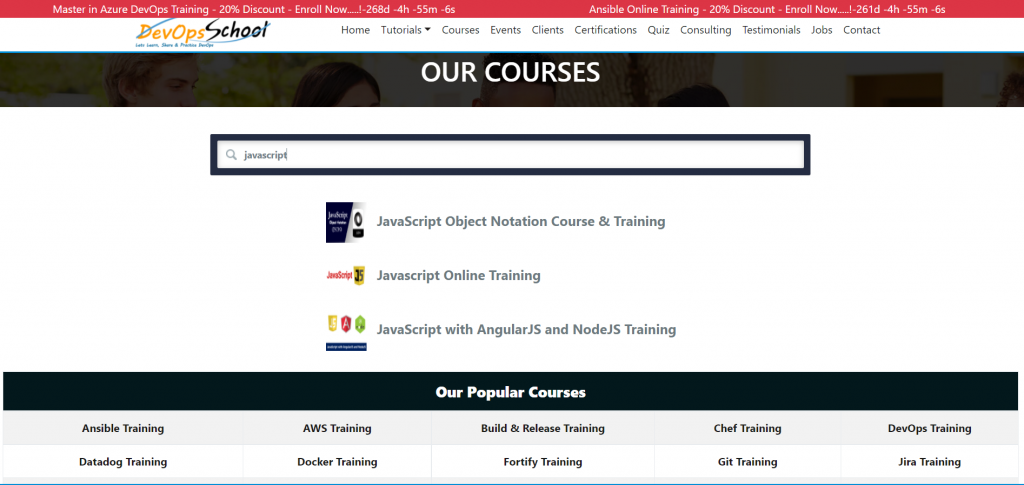A screenshot from the DevOps School website prominently features a dynamic design with swooshy blue lines set against a clean white background. The words “DevOps” and “School” are distinctly colored in vibrant orange and bold black fonts, respectively. The header announces a "Master in Azure DevOps Training" with an enticing "20% discount, enroll now" offer. An embedded countdown timer prominently displays "268 days, 4 hours, 55 minutes, and 6 seconds" remaining. 

Additional training promotions, including "Ansible online training," are highlighted with similar discount incentives. A navigation menu includes clickable links labeled 'Home,' 'Tutorials,' 'Courses,' 'Events,' 'Clients,' 'Certifications,' 'Quiz,' 'Consulting,' 'Testimonials,' 'Jobs,' and 'Contact.'

Further down the page, a semi-transparent rectangular section faintly displays what appear to be the tops of three people's heads in the background, overlaid with the phrase "OUR COURSES" in bold, white, capitalized letters. Below this section is a search bar labeled "JavaScript," followed by a list of course offerings: "JavaScript Object Notation Course and Training," "JavaScript Online Training," and "JavaScript with AngularJS and Node.js Training."